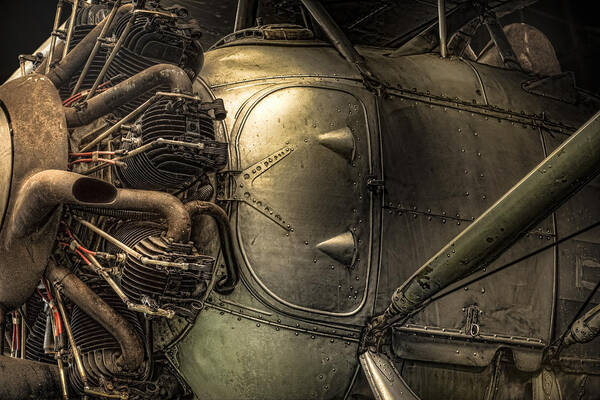This detailed color photograph showcases a vintage radial engine and fuselage from what is likely an old biplane, such as a Douglas C-47 Skytrain. The engine, positioned prominently on the left side of the image, features an array of pistons radiating around it, with metallic pipes and starter wires visibly connected to various radiators. This radial engine is adorned with a rusted patina on its exhaust area, adding to its aged character. The aircraft’s fuselage, seen on the right, boasts a silver metallic surface dotted with metal rivets securing its panels. Visible struts suggest the presence of wings, though they remain outside the frame, and a hint of the cockpit or its windshield is discernible in the upper right corner. The background of the image is black, which starkly contrasts with the polished metallic and aged patina elements, emphasizing the intricate machinist details of this aircraft relic.